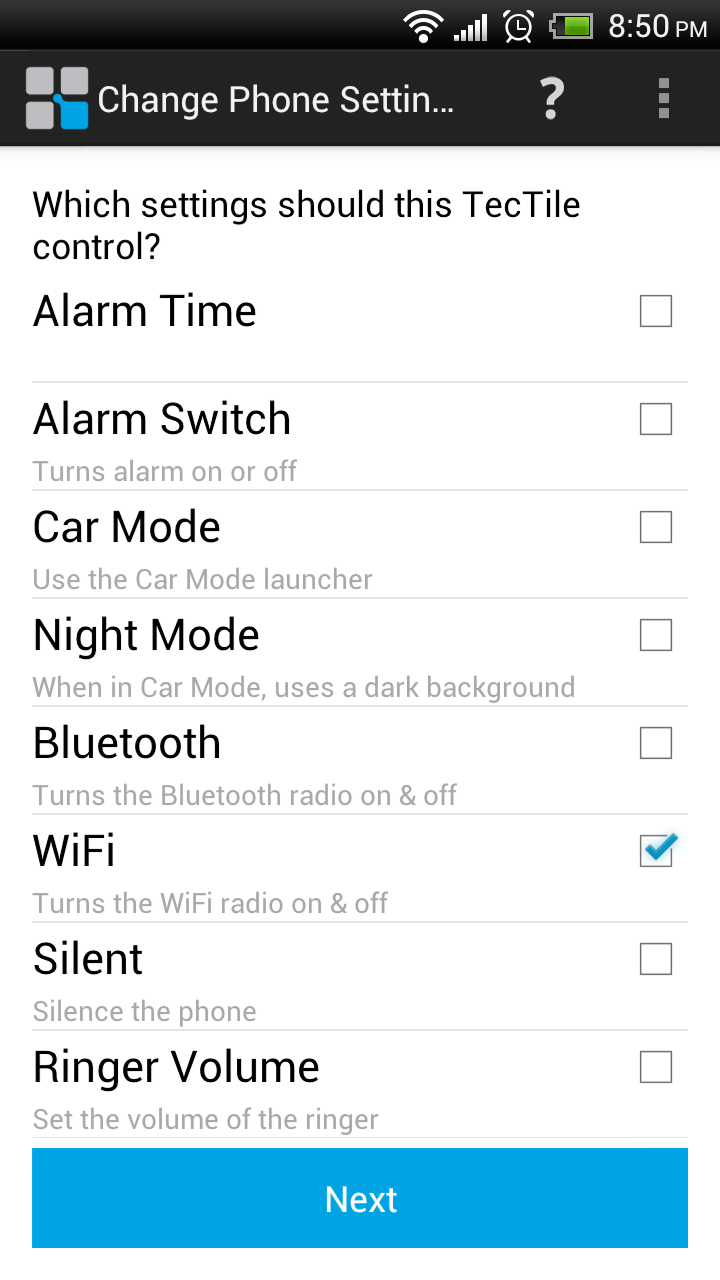At the top of the screen, there is a black border displaying a fully-connected Wi-Fi icon with five bars, an alarm clock icon, and a battery indicator showing approximately three-quarters full. The time is indicated as 8:50 PM. Below this black border, there is a gray area with three gray squares and one blue square, alongside the text "Change Phone Setting?" followed by an ellipsis (...).

Beneath this gray area, on a white background, the text reads: 

"Which setting should this tactile control?"

Below this question, a list of options is provided:
- Alarm Time: Set the alarm time.
- Alarm Switch: Turn the alarm on or off.
- Car Mode: Use the car mode launcher.
- Night Mode: When in car mode, use a dark background.
- Bluetooth: Turn the Bluetooth radio on and off.
- Wi-Fi: Turn the Wi-Fi radio on and off.
- Silent: Silence the phone ringer.
- Volume: Set the volume of the ringer.

There is a blue checkmark next to the Wi-Fi option, indicating it is selected. At the bottom of this list, there is a blue box with the text "Next."